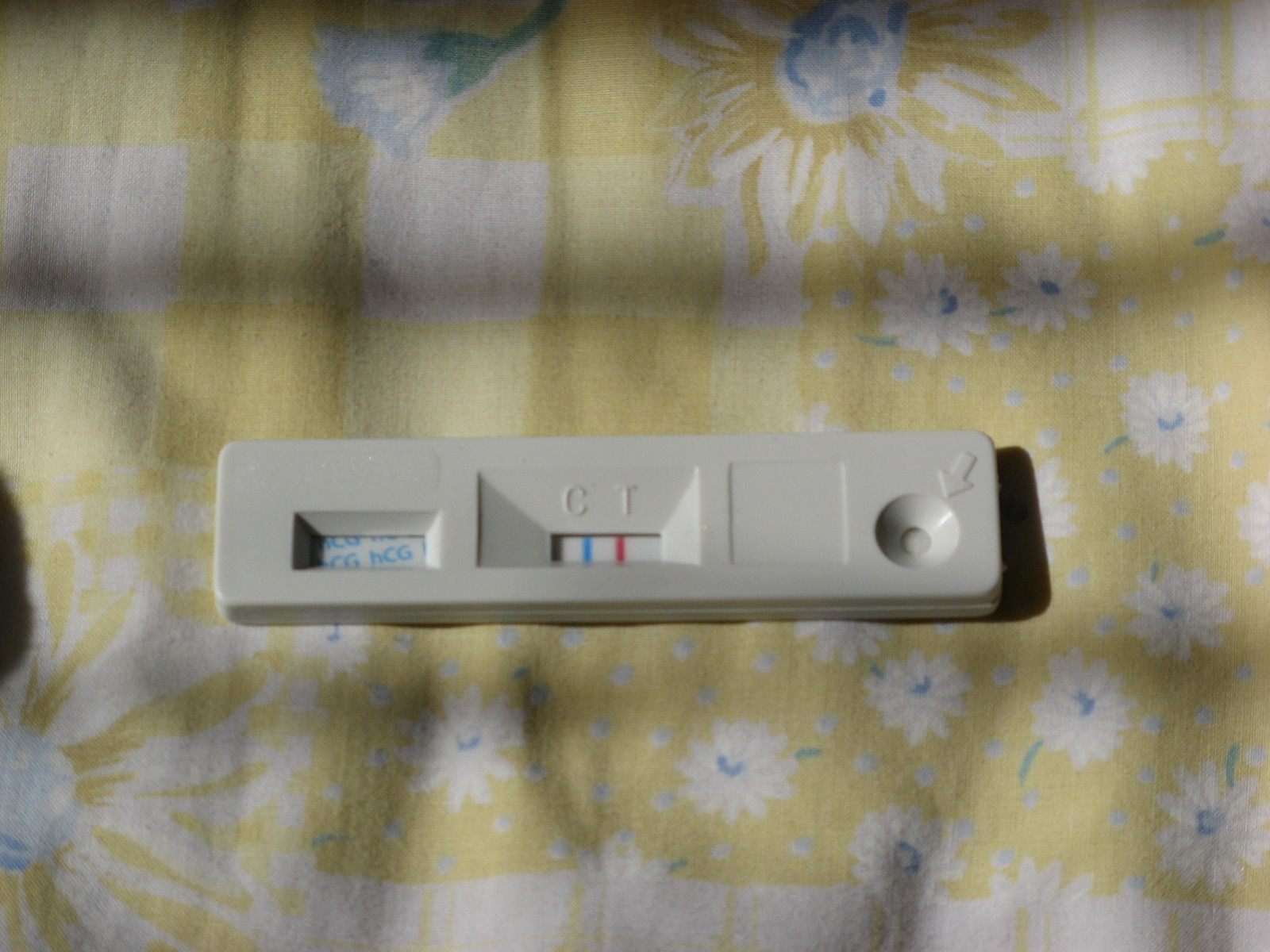This is a detailed photograph of a small white plastic medical test device. The test is resting on a yellow checkered fabric adorned with white and blue floral patterns. The fabric features large flowers, one located in the upper right corner and another in the lower left, while smaller flowers are scattered around the right and lower portions. The yellow checkered pattern consists of two shades of yellow and white, and a white strip runs along the bottom edge of the fabric. The fabric also displays gray horizontal shadows and vertical wrinkles.

The test device itself is a rectangular white plastic piece, approximately five to six times wider than it is tall. On the right side, there is a round indented section indicated by an arrow, designed for a finger press to obtain a blood sample. The central portion has a recessed area labeled "C" and "T", containing a screen that shows a blue vertical bar under the "C" and a red vertical bar under the "T". There is also a smaller screen on the left side of the device, displaying the text "HCG" in blue repeated across a white background. The device does not specify what it tests for but appears to be a finger-prick blood test, most likely for home use.